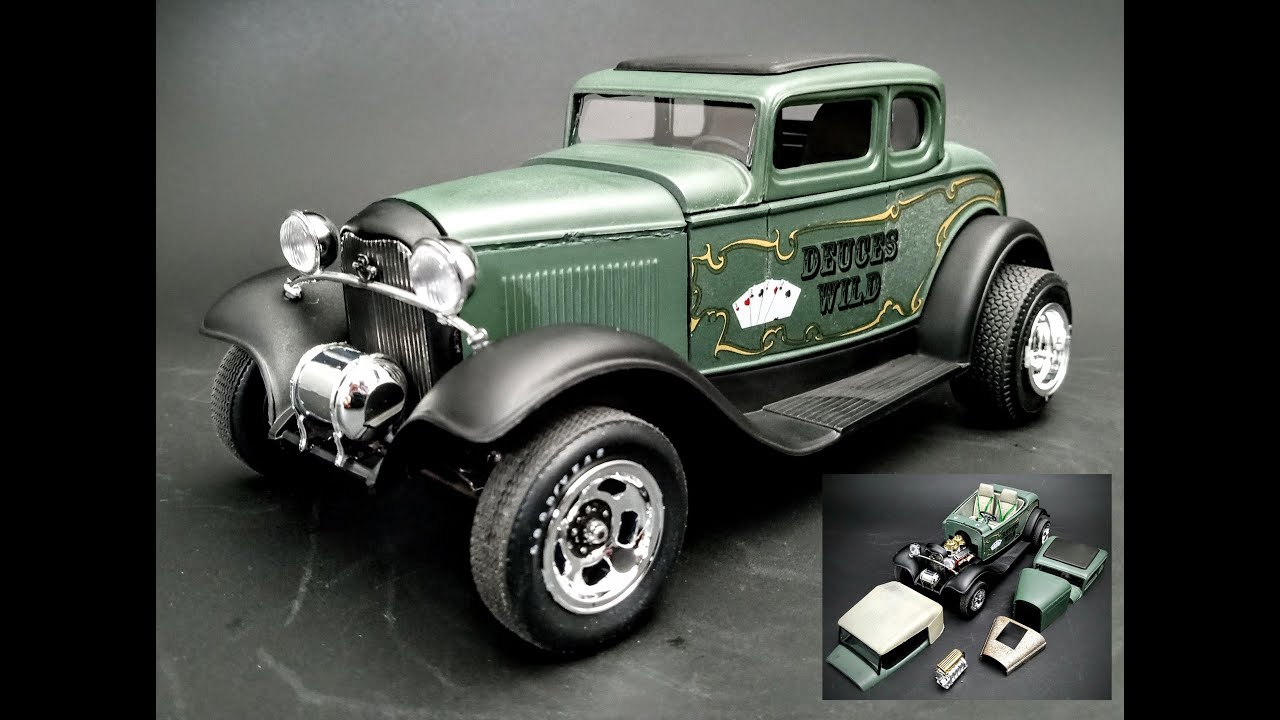This close-up photograph captures a detailed view of a green, vintage-style toy roadster reminiscent of a 1930s Model T. The car is constructed out of shiny plastic, noticeable in the sheen of its faux alloy wheels. Named "Deuces Wild," the car prominently features this title in black text on the side door, accompanied by a small illustration of four playing cards. The toy also includes painted details like black fenders and black baseboards, with a chrome headlight housing and grille. The front of the toy car showcases a tow winch, adding to its rugged, old-fashioned aesthetic. The bottom right corner of the image reveals a deconstructed view of the same model, with various components such as the roof, hood, and engine parts displayed separately. The professional style of the photo suggests it may be used to promote this detailed and well-crafted model toy.